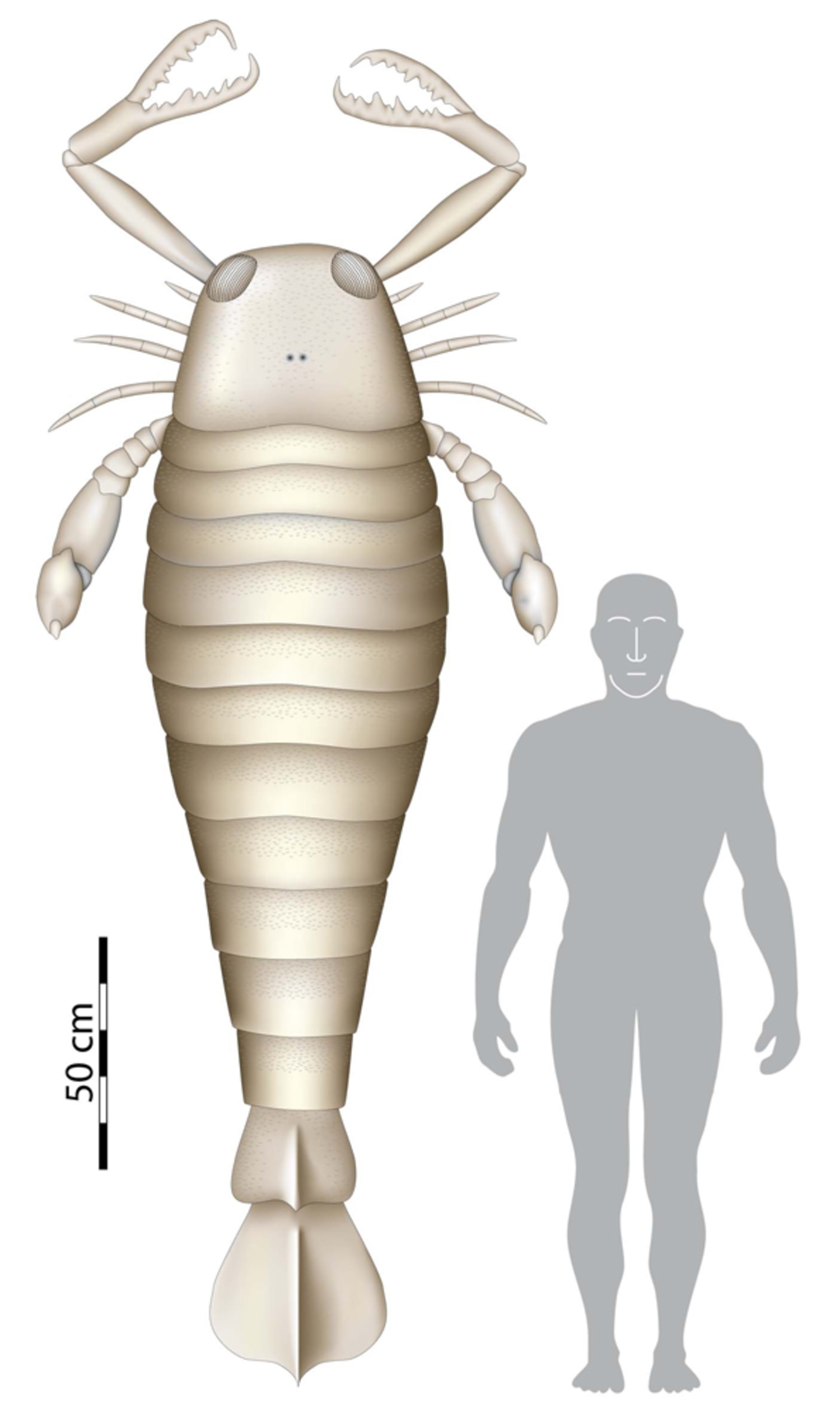The image depicts an animated drawing of a giant crustacean resembling a lobster, standing upright next to a simplified gray silhouette of a human figure on a white background. The crustacean is significantly taller than the human, towering over it by 50 to 60%. Its body is predominantly golden-gray and segmented horizontally, featuring two large jagged-edged pinchers at the front, visible eyes, and two openings on the top of its head. Additionally, it has eight smaller legs positioned off to the sides and two larger, segmented limbs with spiked nubs behind them. The tail of the crustacean resembles a medieval mace, enhancing its fearsome appearance. To the left of the image, there is a size key labeled "50 centimeters," underscoring the substantial size difference between the crustacean and the human figure.